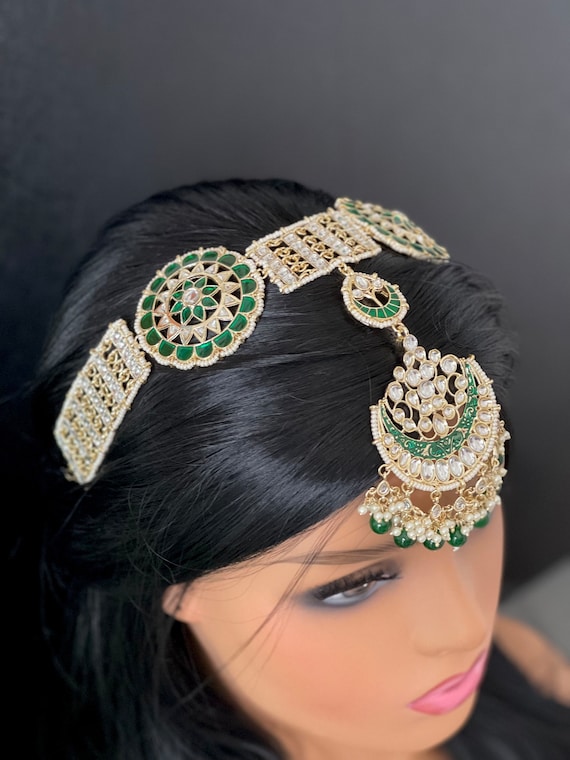The image showcases an elaborately decorated Indian-inspired head ornament adorning a female mannequin's head. The mannequin, with jet black hair and a fully made-up face featuring long eyelashes and pink lipstick, wears a highly detailed piece of jewelry. The headpiece, primarily made of gold, is adorned with diamonds, emeralds, and pearls, extending from the top of the head down to the forehead. The headband itself is composed of intricate segments, including two rectangular shapes and one circle. Emerald and diamond-encrusted circular patterns are positioned on the top left and right sections of the headband, with teardrop green emeralds arranged in a symmetrical design. A crescent-shaped ornament featuring pearl elements is attached to the headband with teardrop embellishments, creating a chandelier-like effect over the forehead. The overall craftsmanship appears handmade, with detailed patterns resembling mosaic tiles from a mosque, enhancing the ornate appearance of the headpiece.